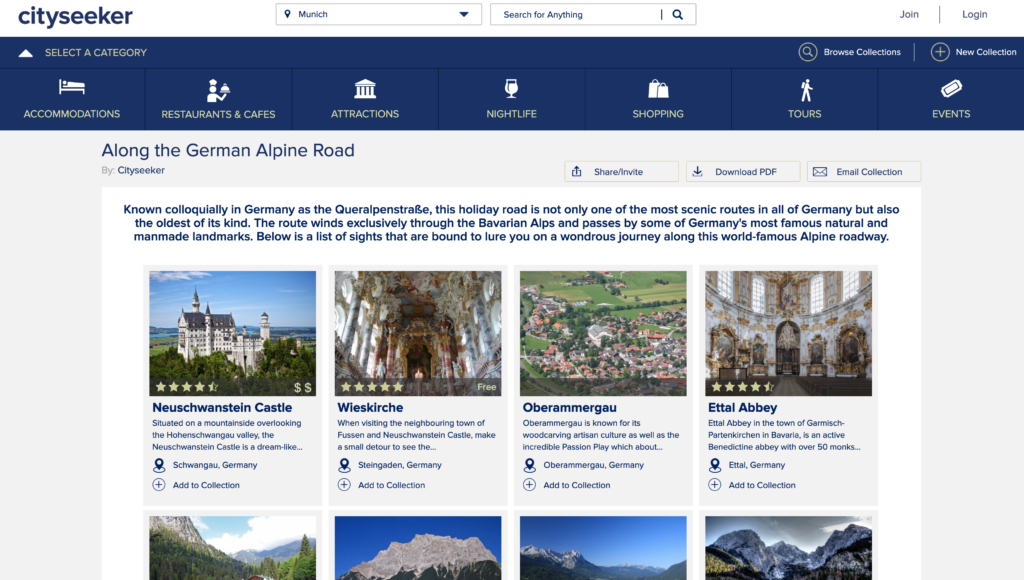The image is a detailed screenshot of the City Seeker website, an online resource dedicated to providing comprehensive information on various attractions, dining establishments, accommodations, and activities within different cities. Prominently featured at the top of the webpage is a search bar, in which the word "Munich" is currently entered, accompanied by a prompt that reads, "search for anything." This indicates where users can input keywords to find specific points of interest within the city.

To the right of the search bar, there are links for users to "Join" or "Log In," suggesting options to create an account or access an existing one. Additionally, a navigation menu spans the top of the page, offering categories such as Accommodations, Restaurants and Cafes, Attractions, Nightlife, Shopping, Tours, and Events, each likely leading to detailed sub-sections relating to those topics.

Beneath the navigation menu, a highlighted section titled "Along the German Alpine Road by City Seeker" captures attention. It explains that the road, known colloquially in Germany as the "Kerlpenstraße", is celebrated not only as one of Germany's most scenic routes but also its oldest. This holiday road meanders through the Bavarian Alps and features some of Germany's most renowned natural and man-made landmarks.

Following the descriptive introduction, the page lists several must-see sites along this world-famous Alpine Roadway. Notable locations mentioned include the fairy-tale Neuschwanstein Castle, the ornate Wieskirche (Church of Wies), the picturesque village of Oberammergau, and Edelabee, each promising to entice visitors on a remarkable journey through this idyllic region.